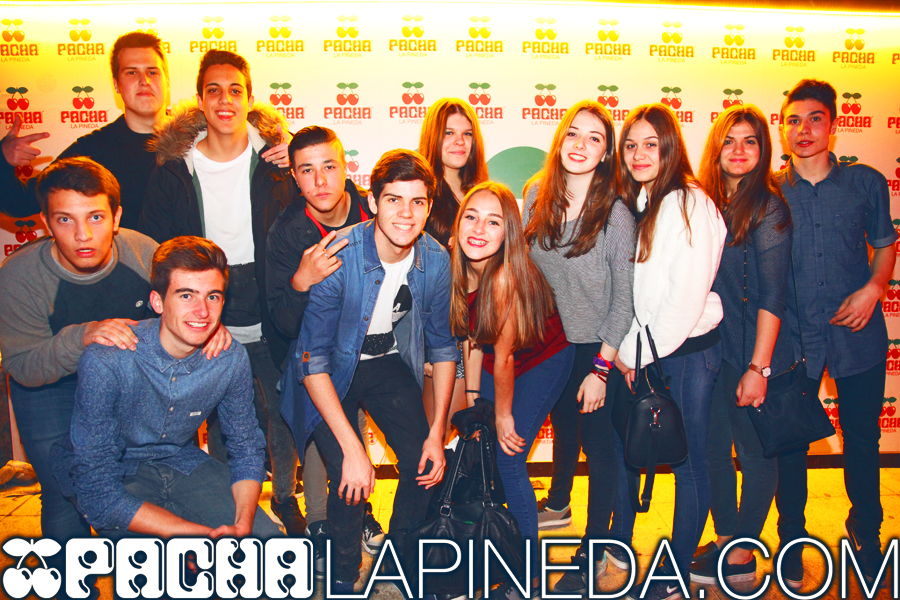The image is a wide-angle photograph featuring a group of 14 Caucasian teenagers, around 15 or 16 years old, posing cheerfully. They are casually dressed, mostly in jeans and a mix of short-sleeved T-shirts and long-sleeved sweatshirts, standing horizontally across the center of the image. At the far left, a young man is crouching down in front of another young man who is also crouching. Moving right, a young man in a white shirt with a fur collar coat stands with a young man in black behind him. Next to them, a young man leans over another crouching young man wearing a denim shirt and white T-shirt, making a playful two-finger gesture. A young woman in a red top with long brown hair leans towards him. Behind her, only the top of another woman's head with brown hair is visible. Adjacent are two young women, one in a grey long-sleeved top and blue jeans and another in a white long-sleeved top with brown hair and blue jeans. Further right is a woman in a blue top and trousers and finally, a young man in a blue shirt and trousers stands at the end. Behind the group, a white wall adorned with a repeating logo featuring two cherries with a single stem, the word "P-A-C-H-A" in red below, spans the background. White text superimposed at the bottom reads "P-A-C-H-A-L-A-P-I-N-E-D-A dot com," accompanied by a cherry silhouette on the left.